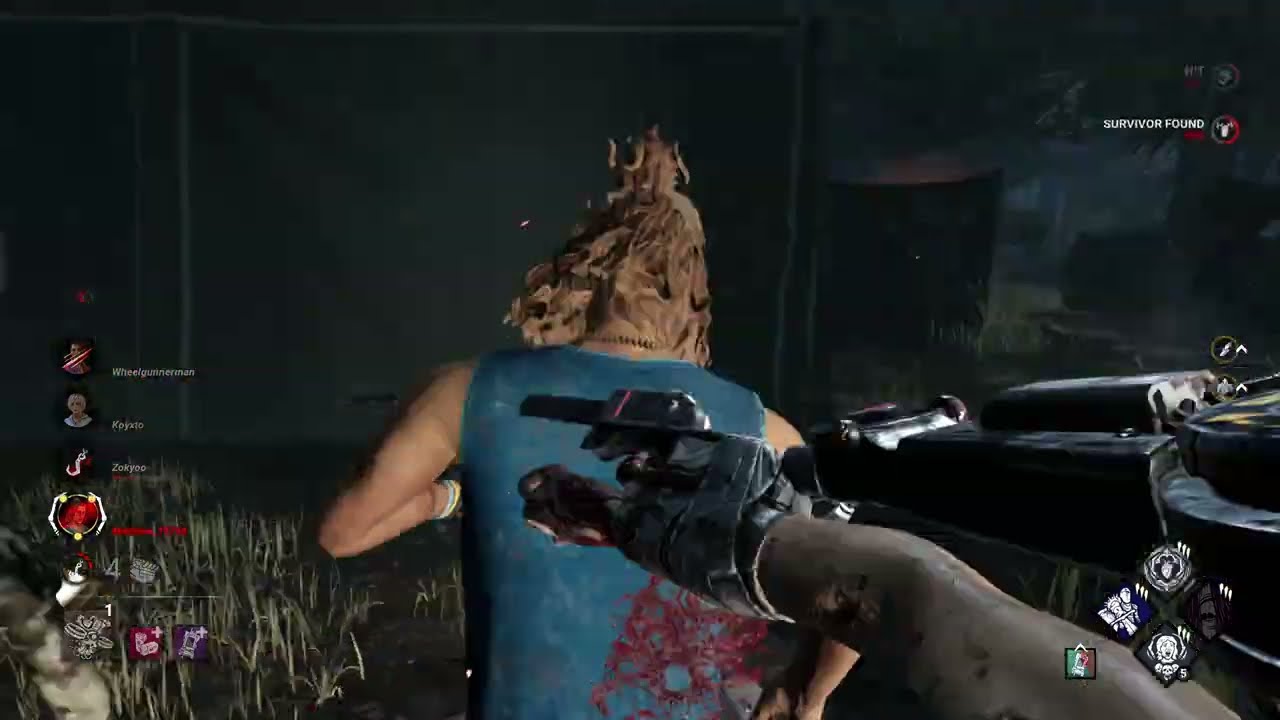The image is a detailed screenshot from what appears to be the game Dead by Daylight, showcasing an intense moment during nighttime gameplay. The perspective is first-person, with the player wielding a makeshift weapon—an arm with a saw blade crudely attached with duct tape, extending from an exoskeleton-like contraption. Central to the image is the back of a blonde-haired woman, her hair tied up into a man bun with long strands draping down. She wears a sleeveless turquoise outfit with a red pattern near the top.

To the right of the woman, an ominous machine with various probes, arms, cylinders, and rectangular objects stands, along with symbols that likely activate its features. Above this scene, an inscription reads "Survivor Found," indicating a key moment in the game. The surroundings are dark and murky, hinting at a tent-like environment with dim lighting. UI elements populate both sides of the screen: player status, health stats, in-game abilities, and additional game information. The lower left corner features low-poly textures of grass and mysterious white fuzzy objects, adding to the scene's eerie ambiance.